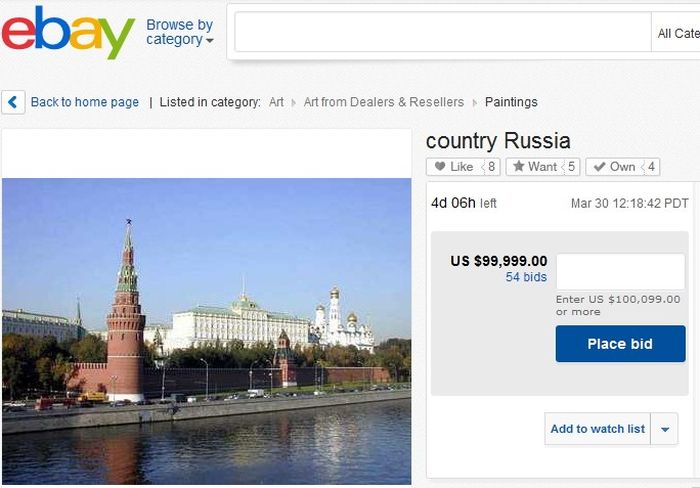**Image Description for Website**

The image has a clean, light gray background. At the top, the eBay logo is displayed in lowercase letters, where the 'e' is red, 'b' is blue, 'a' is yellow, and 'y' is green. To the right of the logo, "Browse by category" is written in blue text, accompanied by a downward arrow.

Beneath this, a white search bar is prominently placed. The search bar shows the incomplete text "all cat", truncated due to the image's cropping.

Below the search bar, a blue square with a white back arrow is present on the left side, alongside the text "Back to the homepage".

Further down, there's a line of black text stating "Listed in category: Art from dealers and resellers > Paintings". The word "Paintings" is in bolder print.

The main section of the image features a photograph with a white background, showing an outdoor scene with a blue sky, water, trees, and buildings. The text accompanying the image includes:
- Country: Russia
- Like: 8
- Want: 5
- Own: 4

Additionally, a white square displays "4D 06H" indicating four days and six hours left in the listing. Below this, it reads "March 30th, 12:18:42 PDT", followed by the price "US $99,999". There are 54 bids, with the option to "Enter US $100,099 or more" for the next bid. Finally, there's a blue square with white text stating "Place Bid".

Overall, the image effectively conveys information about an eBay listing under the Art category for paintings, with detailed bidding and timing information.